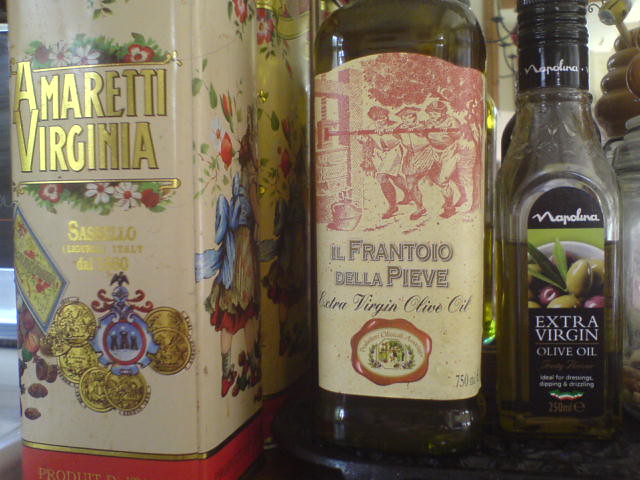This image features a close-up view of three different containers of olive oil, partially cropped at the top and bottom, and slightly blurry but detailed enough to identify the labels. On the left, there is a tan and red tin labeled "Amaretti Virginia" featuring floral designs in gold, white, blue, brown, and cream. The tin's lettering includes "Sessilio, Italy" and other unreadable text. The middle container is a bottle labeled "Il Frantoio della Pieve, Extra Virgin Olive Oil." Its cream-colored label depicts three women, or chefs, pressing olives in red ink, with additional text of "750 ml" at the bottom. Lastly, the rightmost bottle is labeled "Napolina Extra Virgin Olive Oil," featuring a black label with "Napolina" written in white, and an image of olives. In the background, a mirror reflects the back of the left tin, enhancing the close-up perspective of the photograph.